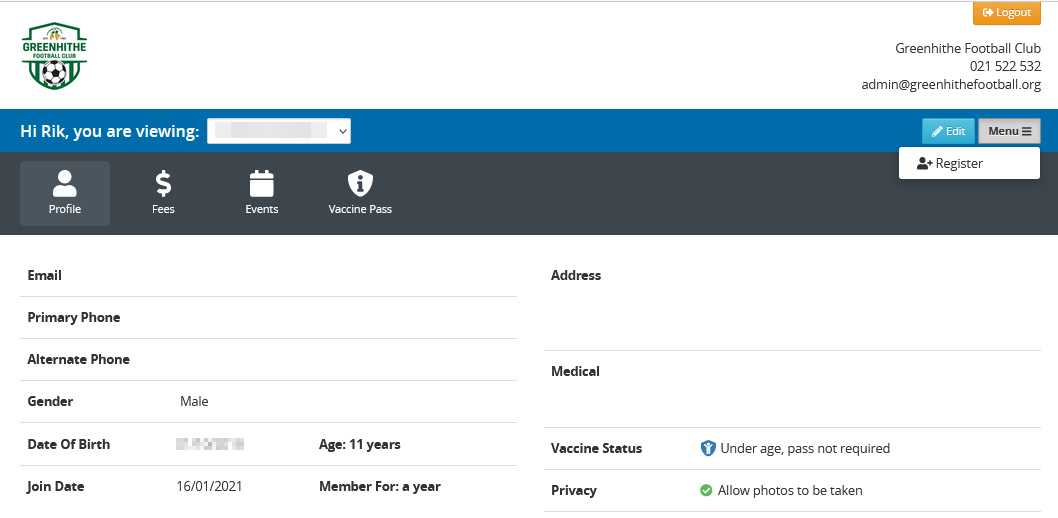The screenshot captures the profile account of a user, presumably Rick, on the Greenhithe Football Club's online portal. In the top-left corner, a green emblem prominently features a soccer ball, along with the club’s name, "Greenhithe Football Club." Adjacent to this, on the right, an orange logout button is visible, displaying an icon of a door with an arrow.

Beneath the emblem, the contact details for the club are listed, including a phone number (021-522-532) and an email address. The entire background of the page is white, with the exception of two text boxes beneath the emblem and email: a blue rectangle and a dark gray rectangle. The blue rectangle contains a blurred message, starting with "Hi Rick, you are viewing..."

The dark gray rectangle serves as a menu with various options such as "Profile," "Fees," "Events," and "Vaccine," with the "Profile" section currently selected. Under the profile tab, detailed information about Rick is listed, including his email, primary phone, alternate phone, gender (male), and date of birth (blurred out). It is noted that Rick is 11 years old and has been a member since January 16, 2021. Additional details provided include his address, medical information, vaccine status, and privacy settings, which are displayed on the right side of the profile.